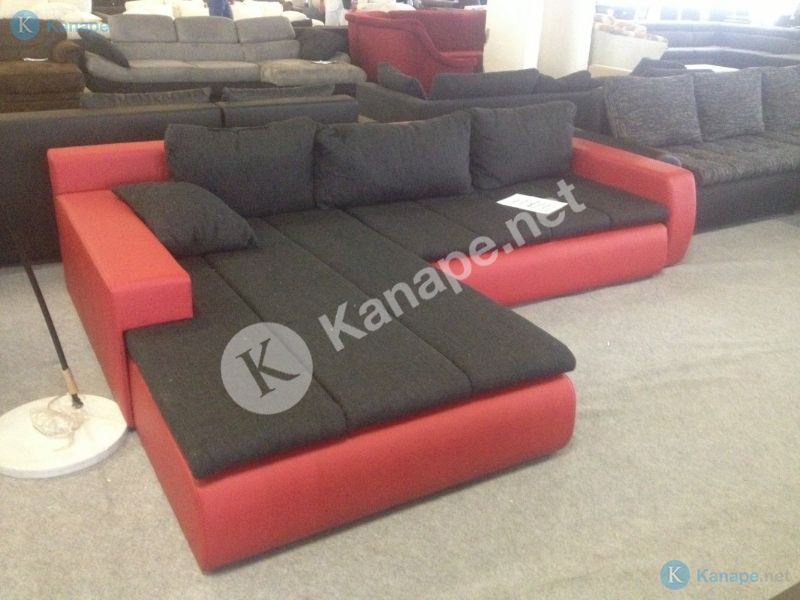The image captures the interior of a bustling furniture store with a light gray carpet covering the floor. Dominating the center of the picture is an L-shaped sectional couch featuring vibrant red leather on the base and sides, contrasting with plush black cushions and pillows on top. The sectional includes a chaise lounge for added comfort. Adjacent to the sectional is a black couch fitted with light gray upholstery cushions. Scattered in the background are various other couches: a three-seater black couch with gray cushions, a brown cushioned couch, a red sofa, and additional black couches placed in a back-to-back arrangement. The scene includes a lamp with a white circular base and a black pole, although its top is cut off in the photo. Prominently displayed over the image is a watermark consisting of a gray circle with a transparent "K" and the text "K-A-N-A-P-E dot net." Additionally, on the bottom right side, there's a blue circle with a white "K" and the text "K-A-N-A-P dot net" in blue and gray.